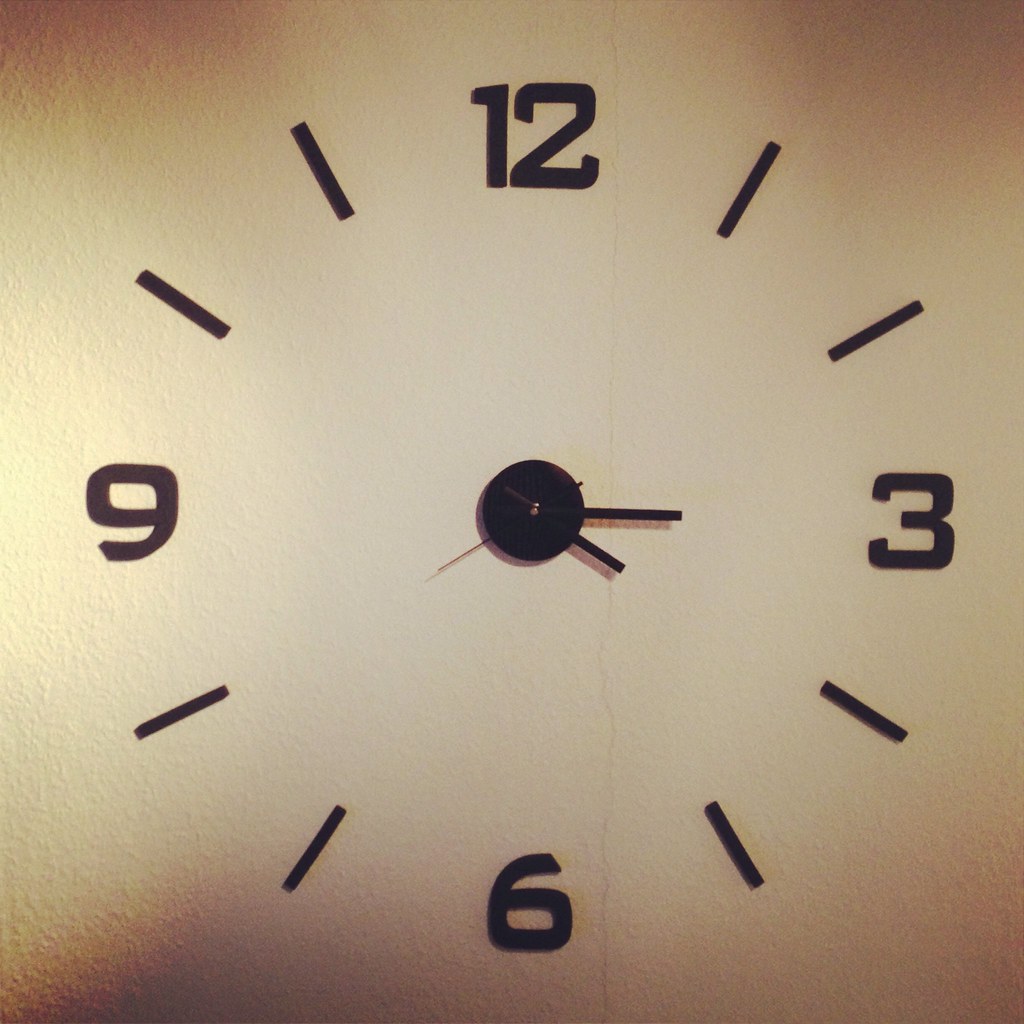This photograph captures a square image of a classic clock face centered in the middle. The background features a subtle brownish gradient that darkens progressively towards each of the four corners, creating a vignette effect. The center of the image is significantly lighter, almost white, drawing the viewer’s attention directly to the clock. The clock face displays large, bold black numbers at the 12, 3, 6, and 9 o'clock positions. Between these numerals are smaller, minimalist tick marks representing each minute, all rendered in black. The clock is equipped with three black hands: one for the hours, one for the minutes, and a thinner one for the seconds. This detailed composition combines elegance and simplicity, highlighting the timeless nature of the clock against the nuanced tones of the background.